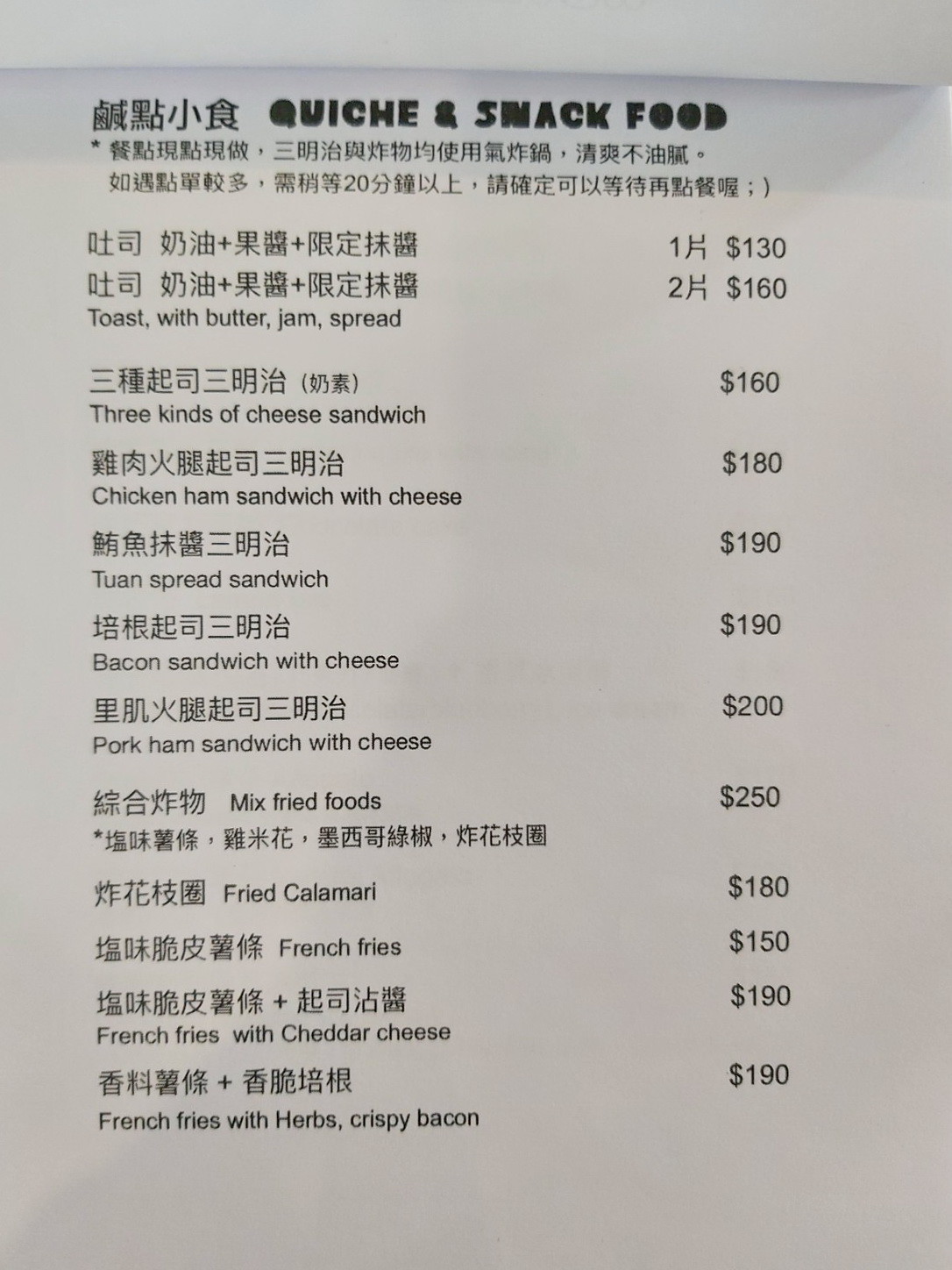A detailed description of the image reveals a menu displayed on a white sheet of paper, likely part of a notepad, as suggested by the rolled edges at the top. The menu features items in both Chinese characters and their English translations. The layout includes the item names listed in Chinese on the left with corresponding prices on the right. Below each Chinese description is the English translation.

At the very top of the menu, bold title text stands out among the numerous instances of Chinese lettering. The menu items and their prices are listed sequentially:

- **Toast with Butter Jam Spread**: $1.30 for one, $1.60 for two.
- **Three Kinds of Cheese Sandwich**: $1.60.
- **Chicken Ham Sandwich with Cheese**: $1.80.
- **Tuan Spread Sandwich**: $1.90.
- **Bacon Sandwich with Cheese**: $1.90.
- **Pork Ham Sandwich with Cheese**: $2.00.
- **Mixed Fried Foods**: $2.50.
- **Fried Calamari**: $1.80.
- **French Fries**: $1.50.
- **French Fries with Cheddar Cheese**: $1.90.
- **French Fries with Herbs Crispy Bacon**: $1.90.

The precise, bilingual presentation of the menu items, along with their affordable pricing, suggests a casual dining establishment or a takeout place offering a variety of sandwiches and fried foods.